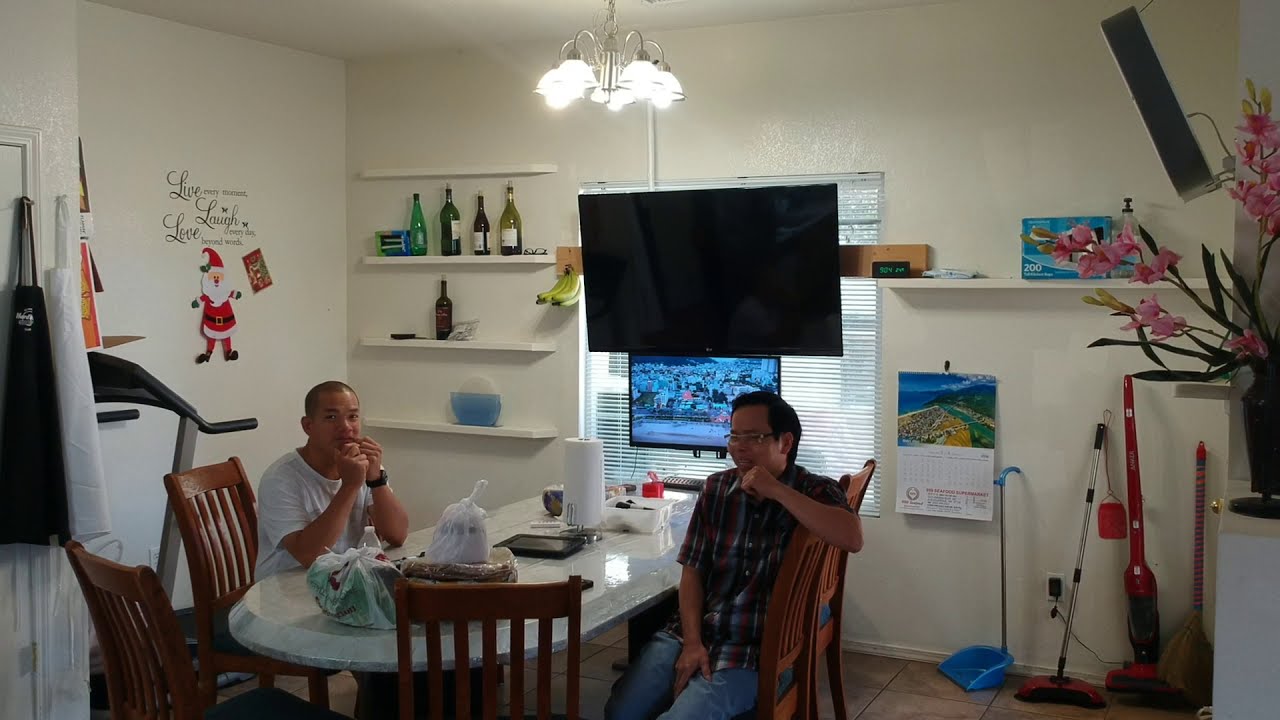The photograph captures an indoor scene in a dining or living area, featuring a white table at the center surrounded by four brown wooden chairs. Two men are seated at the table, one with a nearly bald head looking towards the camera, and the other with longer black hair and glasses looking away. The table is cluttered with takeout boxes, paper towels, and assorted accessories. Behind them, white-painted walls adorned with posters, shelves holding various items including bottles, cleaning supplies, and a calendar can be seen. A figurine of Santa suggests it is Christmas time. Additionally, a TV is mounted above a window, with both a smaller, active monitor displaying content and a larger, inactive TV screen visible. To the left side, there is a wine rack, a treadmill, and a stack of bananas on a rack. In the top center, a chandelier hangs. This detailed setting offers a glimpse into a lived-in and multifaceted domestic space.